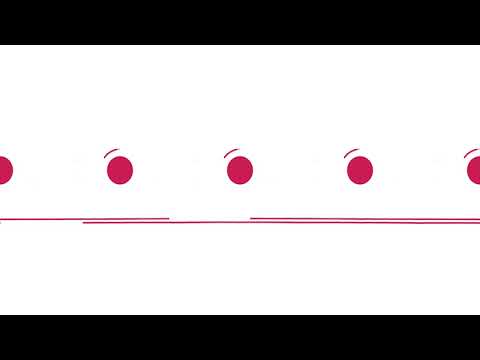The image is an abstract art piece characterized by minimalist design and stark color contrasts. The background is predominantly a grainy white, creating an empty, blank space that serves as a canvas for the distinct elements layered on top. Across the top and bottom of the photograph, there are wide horizontal black bars stretching from left to right. Central to the image, a series of five equally spaced pinkish-red circles runs horizontally. Flanking these circles on the outer edges are semicircles, creating a continuous flow from left to right. Above each circle, there's a small pink curved line that follows the curvature of the circles but does not form a complete loop. Below this sequence of circles, two rows of thin pink horizontal lines are spaced closely together, each line segment interrupted by small breaks. This combination of geometric shapes and lines within the central white rectangle contrasts sharply against the grainy, textured white background, drawing attention to the simple yet intriguing abstract design.